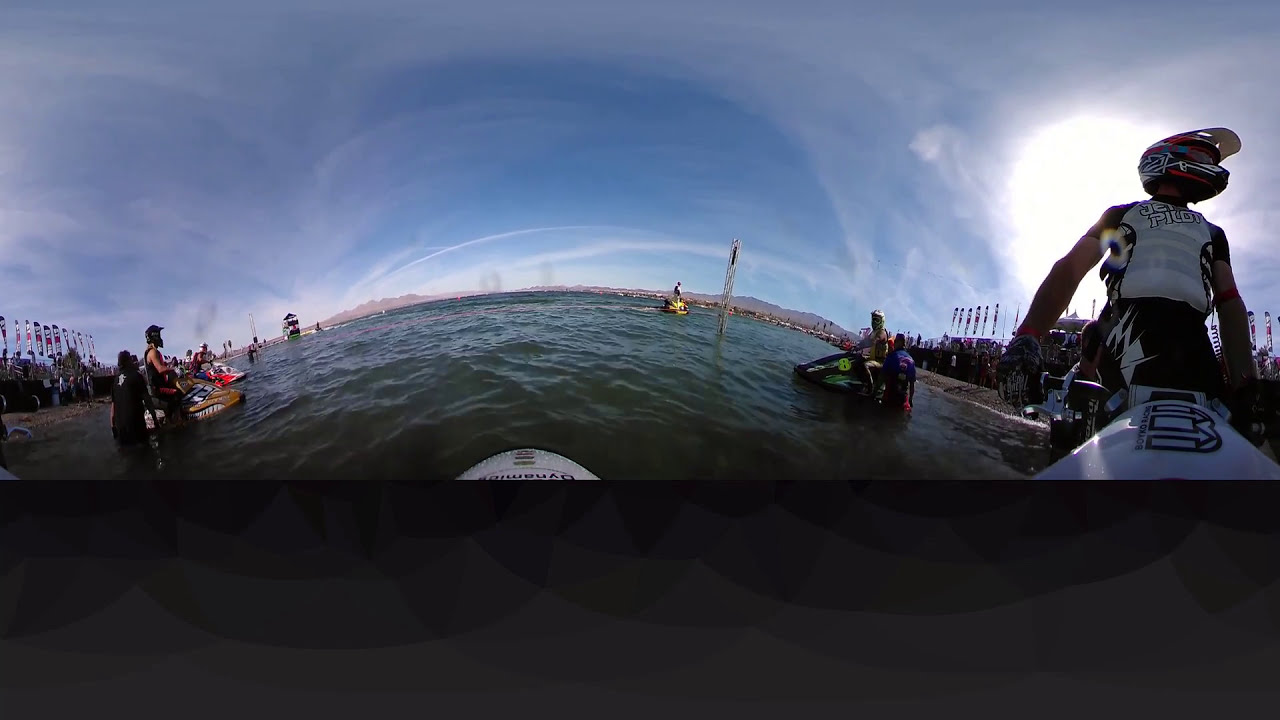In this fisheye, convex image capturing a lively jet ski event, the scene is framed with a black and gray bottom section which gives way to a vibrant, action-packed waterway. The sky, a brilliant blue dotted with clouds, arcs dramatically due to the fisheye effect, emphasizing the curvature of the horizon. To the right, a man rides a white wave runner, donned in a white life vest, black pants, gloves, and a red and black helmet, gripping the throttle while standing. Behind him, spectators watch from stands lining the shoreline. Flags and banners suggest an organized race, with numerous jet skis occupied by riders dressed in a mix of long-sleeved uniforms and tank tops. The choppy, dark waters reflect the bright sun, splitting into shallow and deeper sections. In the background, rolling hills and distant buildings curve upwards, enhancing the sense of a panoramic view. The left side of the image shows more jet skis with riders waiting, flanked by the shoreline, contributing to the dynamic and competitive atmosphere of this water sport event.